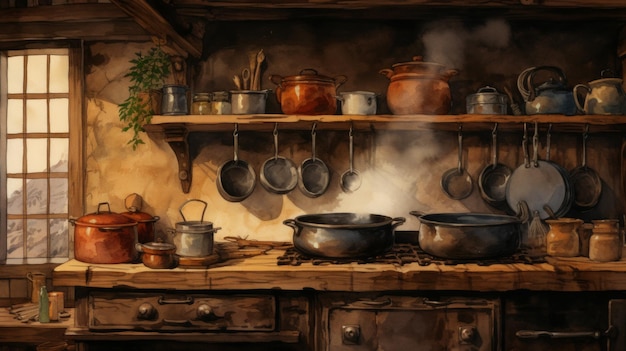The image depicts a highly detailed painting or digital representation of a rustic kitchen, likely in a wooden house or hut. The kitchen is bathed in daylight, streaming through a rectangular window on the left, framed with wooden borders, and offering a glimpse of distant hills. The room's walls and ceiling are composed of wooden planks, creating a warm, earthy ambiance.

Central to the composition is a long, light brown wooden countertop that also functions as a stove. Below the countertop, several dark brown drawers are visible. Positioned on the countertop are different sized pots—specifically, a large red pot, a silver pot, and a smaller red pot on the left side. Centered on the stovetop are two shallow silver pots, with the one on the left emitting a significant amount of steam.

On the right side of the countertop, a series of brown canisters are neatly arranged. Above the countertop, a lengthy wooden shelf runs the span of the wall, cluttered with various cookware, including multiple silver pans, pots, and a green vine adding a touch of nature. Pots and pans hang from hooks attached to the bottom of the shelf, showcasing a combination of functionality and rustic charm.

This meticulously depicted kitchen scene evokes a sense of warmth and homeliness, capturing the intricacies of culinary tools and the inviting atmosphere of a well-used, loved kitchen space.